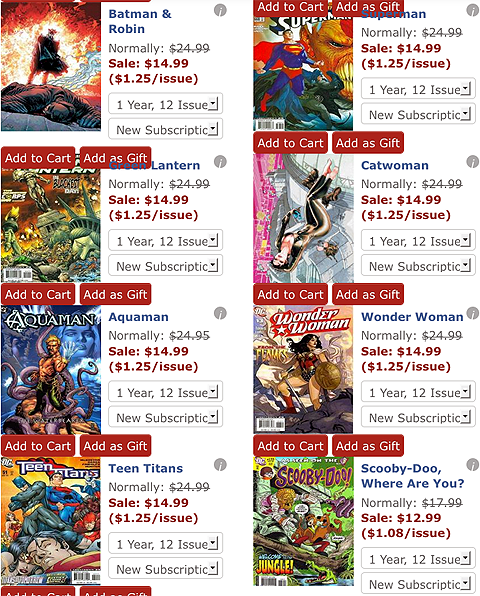The image showcases a page featuring various comic books for sale. 

In the top left corner, there is a slightly blurry picture depicting a caped figure standing against a fiery background, with another figure lying on the ground in the foreground, likely Batman. The comic is titled "Batman and Robin," with the original price of $24.99 crossed out and a sale price of $14.99, equivalent to $1.25 per issue for a one-year, 12-issue subscription.

Below this, another comic book cover is displayed, featuring the head and torch of the partially destroyed Statue of Liberty. This comic is titled "Green Lantern," also priced originally at $24.99, with a sale offer of $1.25 per issue.

Adjacent to it is a comic book cover of Aquaman entangled in a mass of tentacles. The title "Aquaman" is next to it, with the price originally at $24.95, now on sale for $14.99, which is $1.25 an issue.

An icon featuring Batman standing beside Superman, with Wonder Woman and other superheroes in the background, is also shown, with its price listed nearby.

In the right-hand column, there is an image of a Superman comic cover, showing Superman in the foreground and Batman behind him. Below this, another cover depicts Catwoman standing on a building. 

The next comic down is titled "Wonder Woman," with an image of her holding her shield. 

Further down, a comic book cover labeled "Scooby-Doo" features Shaggy and Scooby-Doo, accompanied by the text "Welcome to the Jungle." Next to it, the comic title "Scooby-Doo, Where Are You?" is on sale for $12.99, translating to $1.80 per issue.